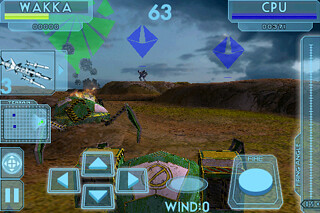The image depicts a detailed screenshot of a video game scene set in a rugged, terrain-like environment, possibly another planet, characterized by a brown, desert-like floor and low mountains under a gray sky. Central to the scene, there is a green and black creature with spider-like legs being shot at, with visible fire emanating from it, indicating missile impact. A white, silver-covered, flying object or satellite approaches from the left side, where a multitude of on-screen displays clutter the edges. These displays include arrow symbols for player movement (up, left, right, down), a pause button, a map navigation symbol, and a missile indicator. Text elements show 'WAKKE' at the top-right in light blue, the number '63' prominently in the center, and 'CPU' also in light blue on the upper-right side. At the bottom of the image, the text 'wind: 0' stands out in baby blue. Additionally, there's a yellow stripe and dot patterns near the top, and smaller details such as blue diamond-shaped figures and the number three are present, adding to the busy, information-dense interface of the game.